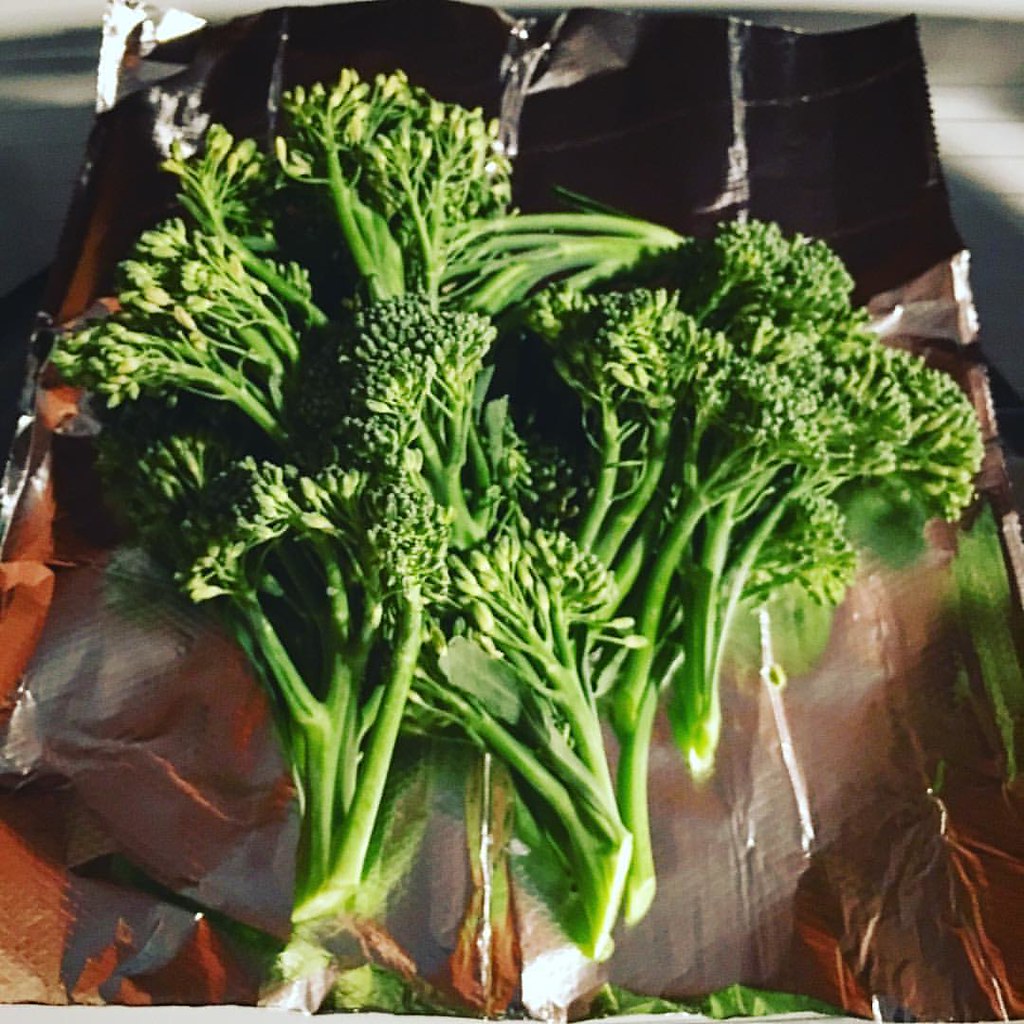The image depicts several vibrant, green, and healthy-looking broccoli florets, some of which resemble broccolini. These florets are arranged closely together—both stacked and laid side by side—on a sheet of aluminum foil. The broccoli appears uncooked and freshly picked. The aluminum foil, featuring some folds and creases, is placed atop a plastic bag that is black with red accents and transparent at the bottom. The background reveals white wooden slats, characteristic of a table, running horizontally across the scene. Ambient light in the somewhat dark room appears to be coming from a window to the right-hand side, adding a subtle natural glow to the broccoli.